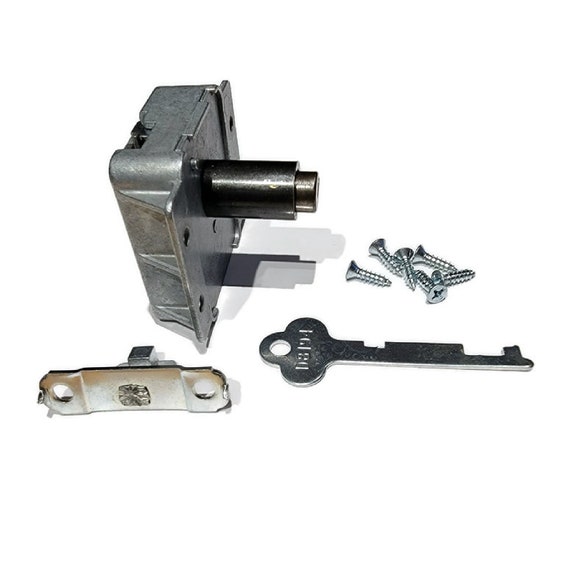A detailed close-up image captures a silver-colored lock and its matching key. The lock itself features a cylindrical back and a square-shaped body. To the left of this sturdy lock is a small rectangular metal bracket, possibly used for mounting. The key boasts a distinctive, clover-shaped top with a hole in it, adorned with some letters. The shaft of the key is elongated and rectangular, featuring two precise notches. Above the key lies a neat pile of six short screws, each with a round head, a central cross indentation, and spiraled threading.